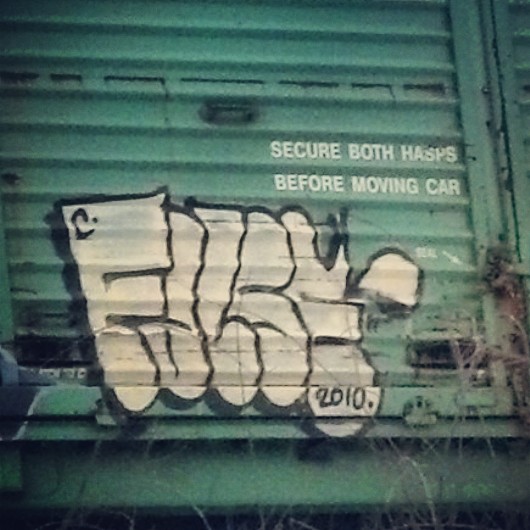The photograph captures a close-up view of a green railroad car, prominently featuring a black-handled door adorned with a combination of official text and graffiti. The focal point is the white, capitalized printed text instructing, "Secure both hasps before moving car." Beneath this directive lies a graffiti tag in white letters with black borders, spelling out "F-O-L-S-E." Notably, the lower part of the final 'E' in this graffiti bears the numerals "2010" in black. The scene is framed by some visible greenery or weeds at the bottom, adding a touch of nature to the industrial setting.